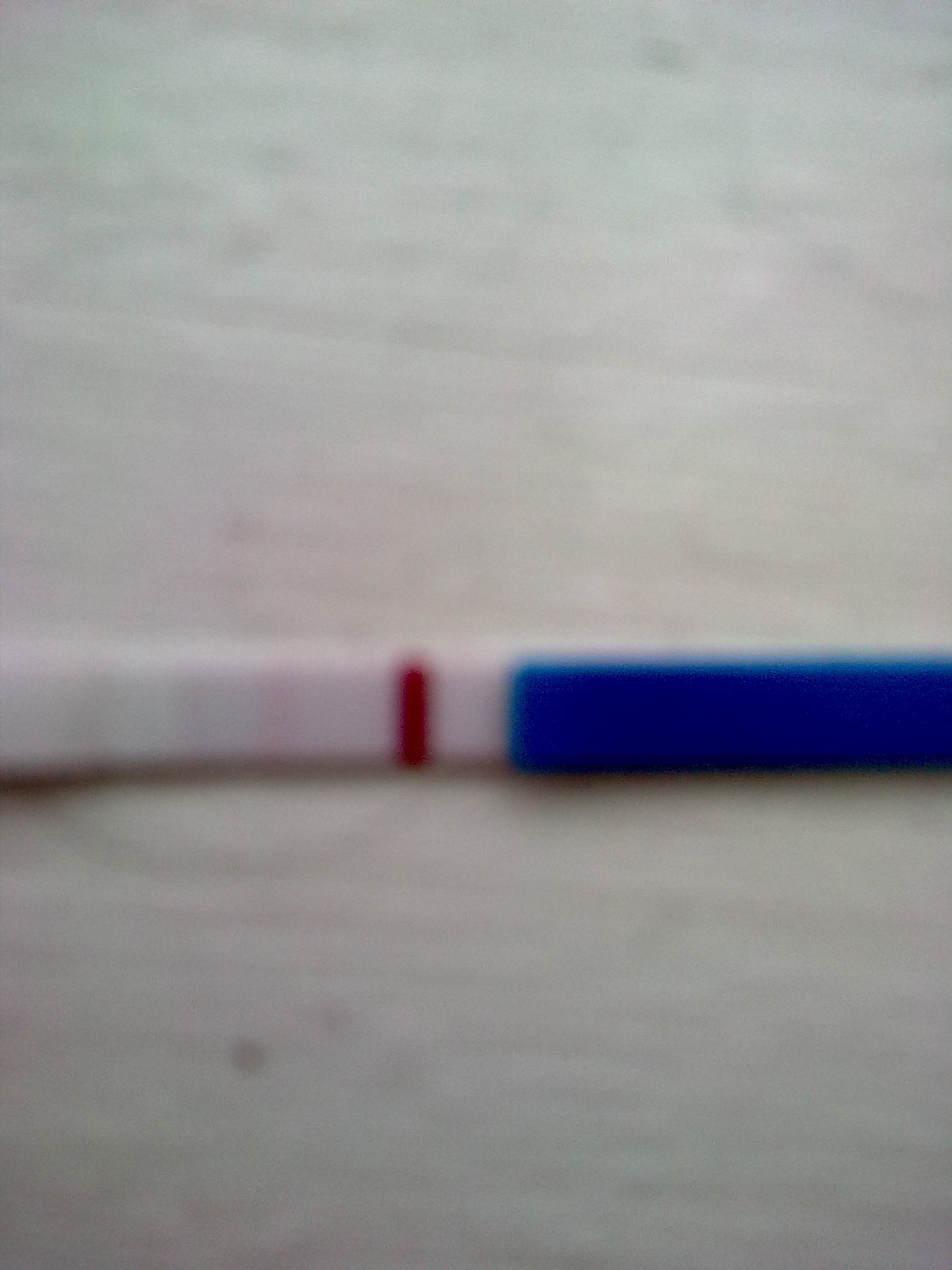This vertical photograph is exceedingly blurry, rendering it difficult to ascertain the subject clearly. The backdrop appears to be a surface resembling gray wood. Positioned on this wooden surface is a horizontal object that spans from the left to the right side of the image. This object is reminiscent of a pregnancy test due to its design. It is a bar segmented into two distinct halves: the left half is white, and the right half is blue. Notably, there is a red line running vertically through the center of the white section, stretching from the top to the bottom of the bar. Despite the lack of clarity in the photo, these details stand out against the indistinct background, suggesting a simple yet recognizable form.